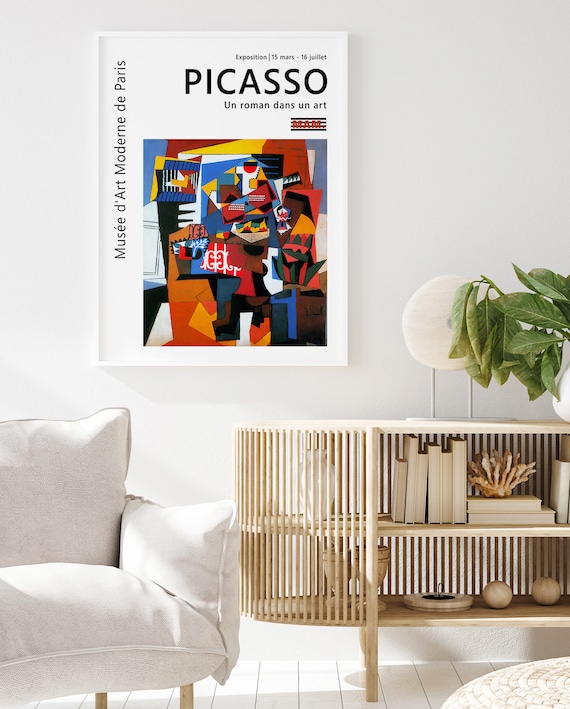In this image of a meticulously designed room, the lower left corner showcases a cozy, white couch adorned with several white pillows, though only the right half of the couch is visible. This couch is supported by elegant, light brown wooden posts. To the right of the couch is a chic coffee table, which is predominantly white with light brown wooden accents. The table features open shelves underneath, filled with various wooden ornaments, including spherical objects, resembling balls, and a few decorative pieces that take the form of small plants and books. Atop the table sits a lush, green plant in a white pot, accompanied by a small white statue.

On the wall above these furnishings hangs an art piece, a tribute to Picasso, inscribed with text in a foreign language. The artwork is an abstract painting, vividly colored with red, blue, yellow, black, and white hues, capturing the quintessential style of Picasso’s work. The room is tastefully decorated, exuding a blend of modern and natural elements through its choice of furniture and artwork.